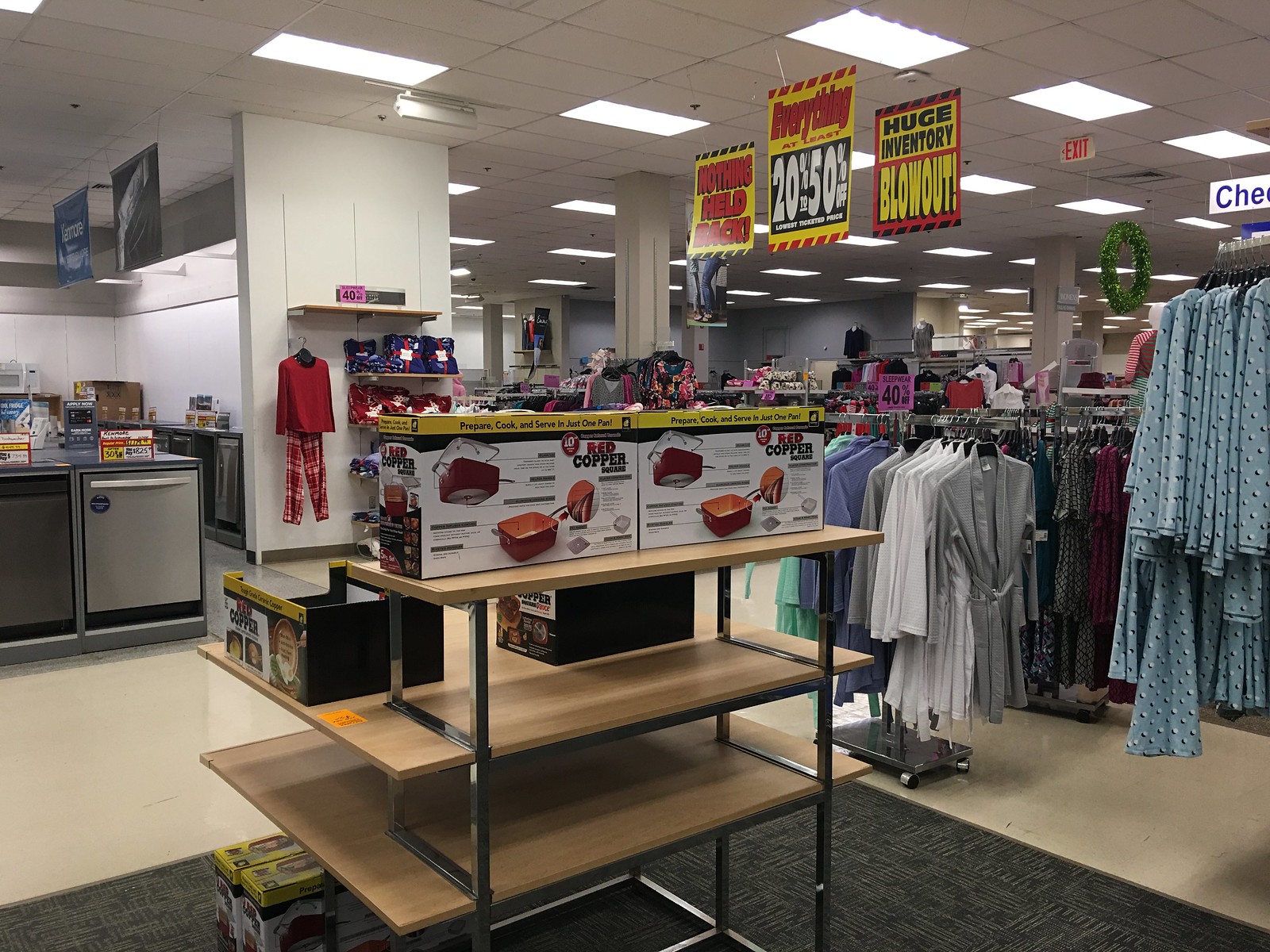This photograph captures a bustling department store from an elevated perspective, providing a sweeping view of the appliance and women's clothing sections. In the foreground, a prominent display of red copper cookware is arranged on a three-tiered rack, surrounded by various other kitchen items. To the left, a row of dishwashers is visible, highlighted by sale tags, indicating their availability.

The women's clothing area stretches out beyond the appliances, distinguishable by racks adorned with items featuring flowery embroidery patterns, bathrobes, and nightgowns. A hint of a children's section can be seen in the background, suggesting a diverse retail space.

Above the merchandise, large advertisement signs catch the eye, declaring a massive inventory blowout sale with discounts ranging from 20 to 50 percent off. The ceiling, typical of a mid-to-late 20th-century department store, is fitted with bright panels and lighting fixtures. An exit sign hangs prominently, guiding shoppers towards multiple directions within the store.

The overall ambiance is reminiscent of traditional American department stores such as Macy's or JCPenney's from the 1990s to 2000s, evoking a sense of nostalgia for an era of extensive in-person shopping experiences.